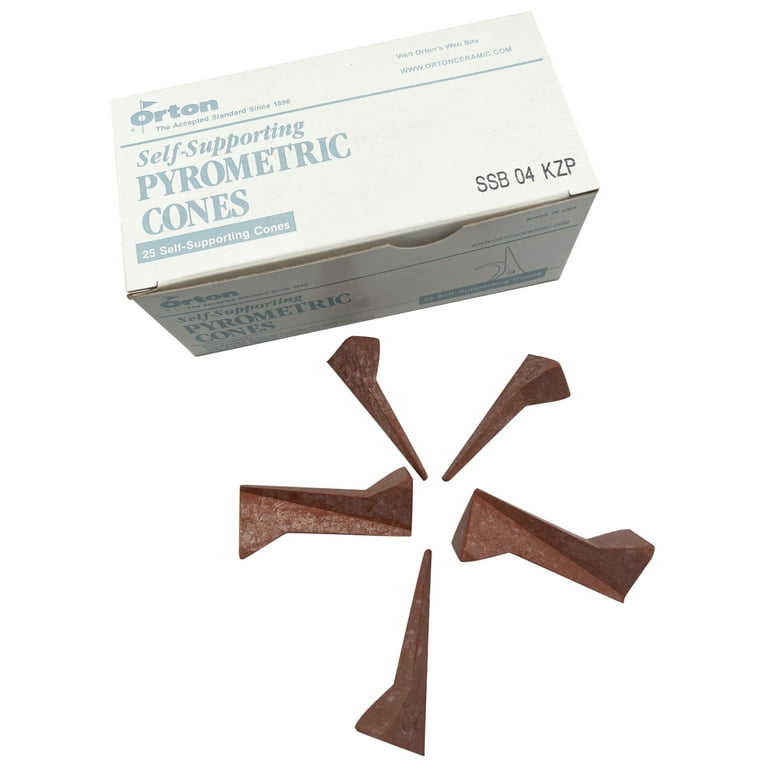In this image, we have a white background highlighting a product display centered around a box and its contents. The off-white box features prominently at the top with the brand name "Orton" written in a faded teal color on the top left corner. Below the brand name, the box is labeled "self-supporting pyrometric cones," with a further description indicating "25 self-supporting cones" on the lower left. Additionally, there is some text "SSB 0 4 K Z P" on the bottom right and a partially obscured website URL with light glare affecting its readability.

The box is closed, but the contents, a collection of brown pyrometric cones, are displayed below it. These cones are meticulously arranged in a star pattern. They exhibit a rusty brown, chocolate-like hue and vary in size and shape; some cones resemble golf tees or spikes, while others are larger, resembling columns or pillars. The detailed presentation provides a clear and engaging view of the product, combining elements from multiple perspectives to offer a comprehensive description.